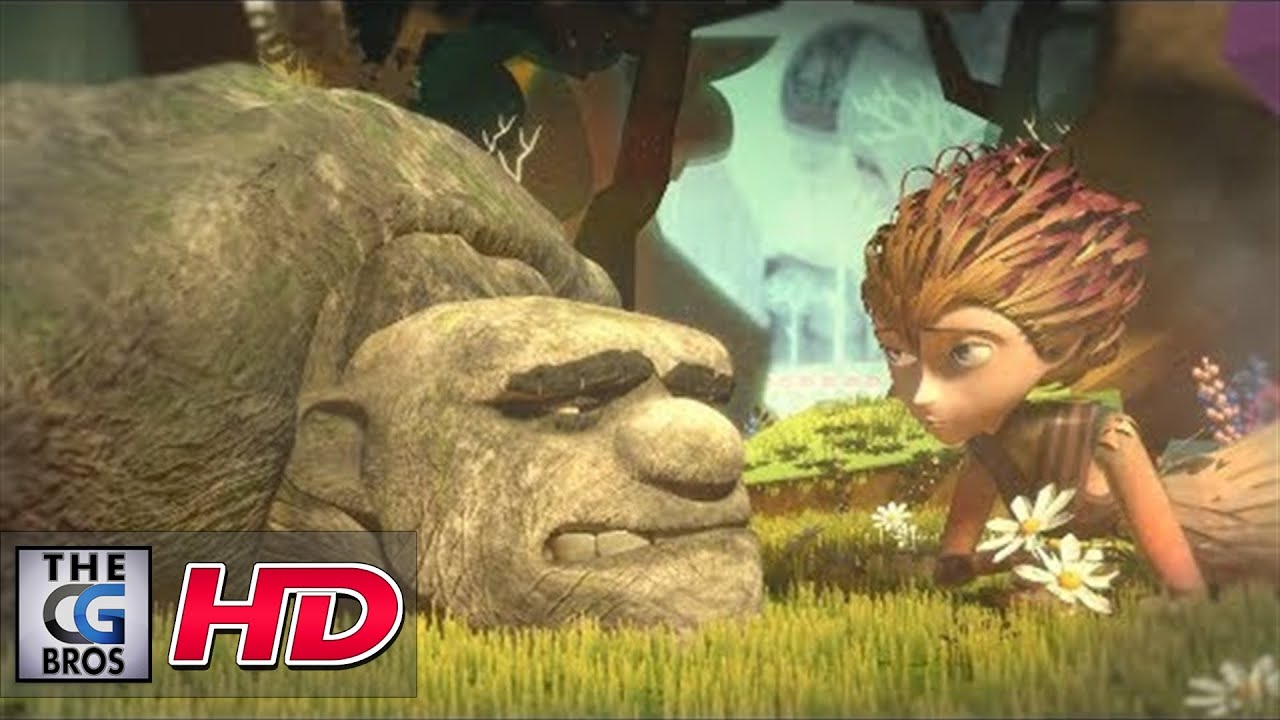This detailed cartoon-style image features a whimsical and touching scene between two fantasy characters laying on a bed of lush, drawn grass. On the left side of the image lies a large, golem-like creature with camouflaged brownie green, thick wrinkled skin. His chin is resting on the ground, and he has a round, bulbous nose with two large exposed teeth. His thick black eyebrows frame a pair of sunken eyes, giving him a somber expression. 

Opposite him, on the right side of the image, is a thin, fairy-like figure with wild, reddish-brown hair swept back, wearing a simple brown dress. She mirrors his pose, lying on her stomach, propped up on her elbows, holding a bunch of daisies close to the grass. Her expression is one of gentle concern as she looks back at the creature.

In the backdrop, a subtle fantasy forest adds layers of depth with soft blues and light hues. The words "The CG Brothers" appear as a logo in a box at the lower left corner, next to a red "HD" logo, tying the image together.